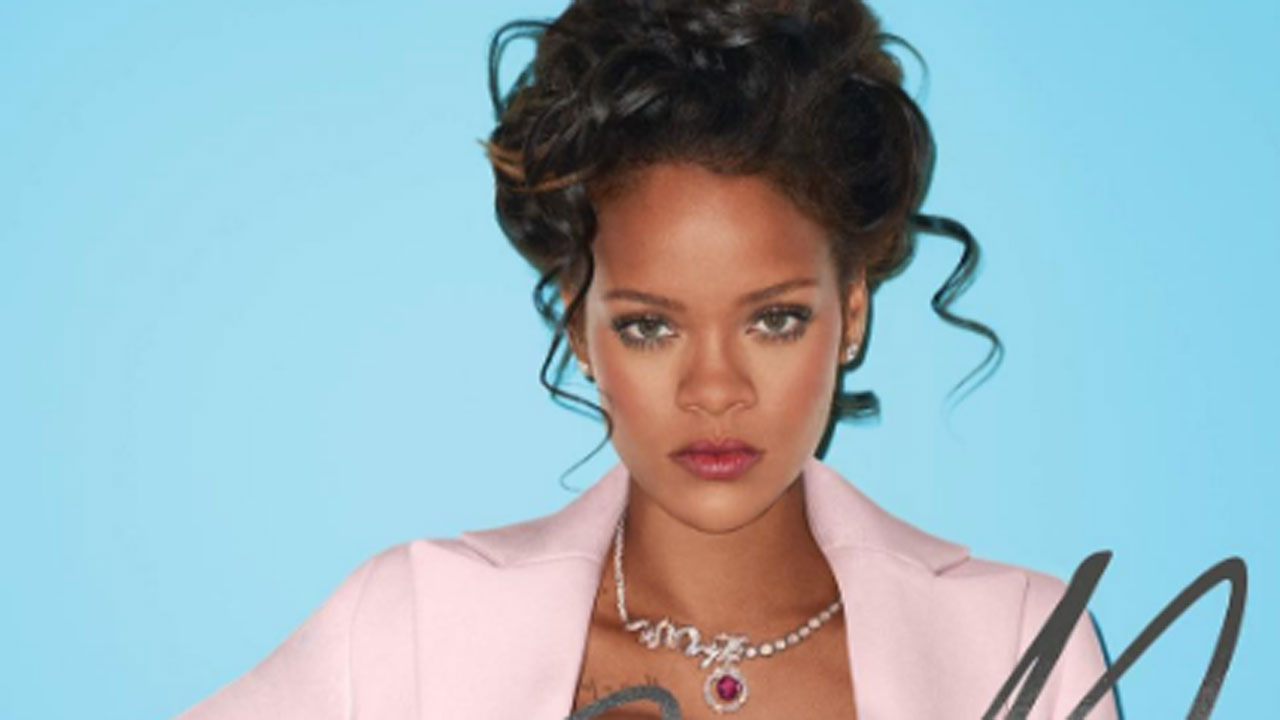The image features Rihanna, known for her distinctive dark complexion and long, dark hair, which she has styled in an elegant updo. Delicate tendrils of hair gracefully frame her face, one on each side. Her makeup is flawlessly applied, enhancing her radiant features. She is dressed in a pale pink blazer without a shirt underneath, giving a bold yet sophisticated appearance. Around her neck, she sports a stunning necklace comprised of diamonds with a central ruby pendant, adding a touch of regal glamour. A notable mark is visible on her chest, which could be a tattoo or a signature spontaneously inscribed on the photo. The backdrop of the image is a light blue hue, providing a serene contrast to her striking ensemble. Additionally, she completes her look with a pair of stylish earrings.